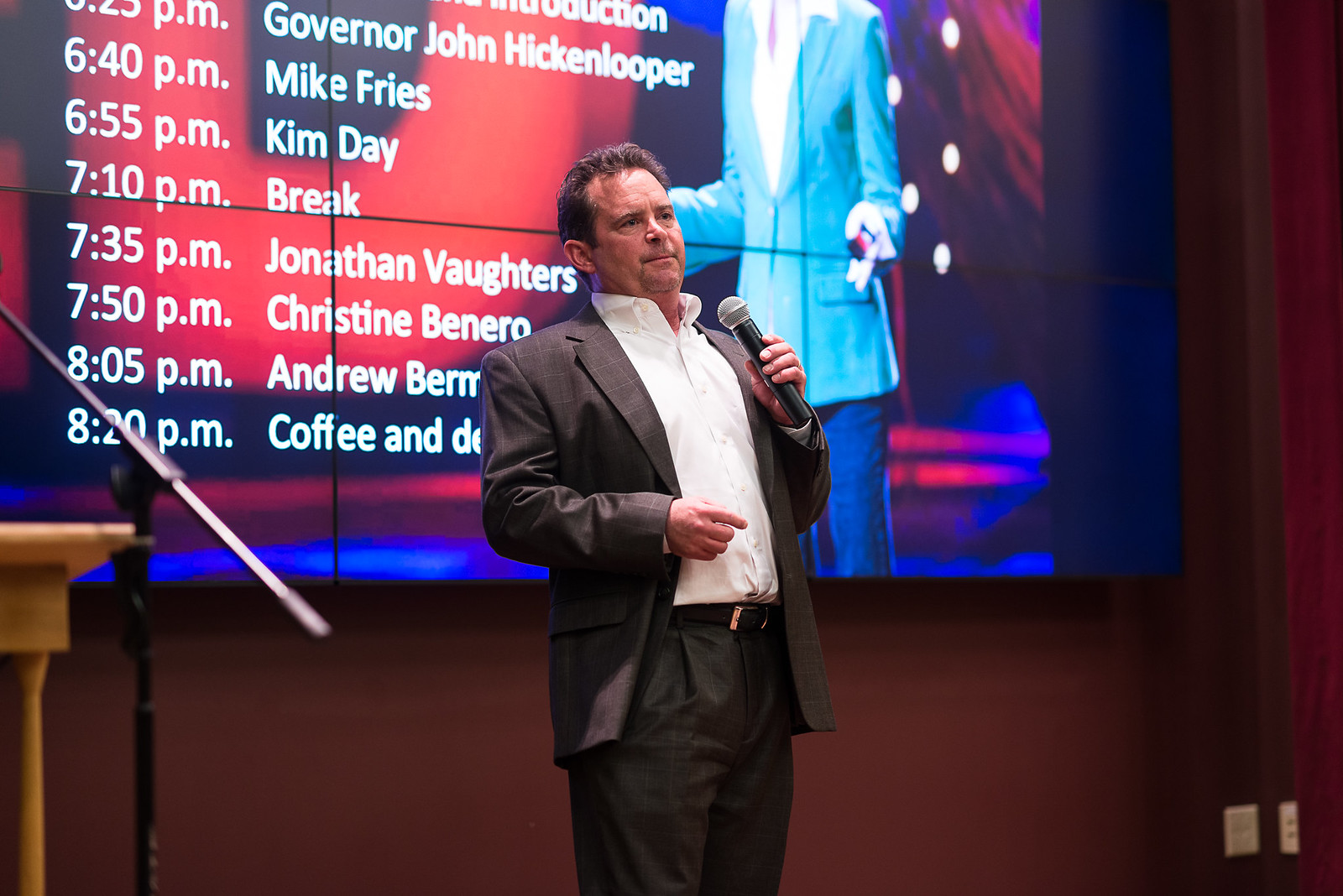A suited man with short brown hair, appearing to be in his late 30s, stands on a stage holding a microphone, seemingly addressing an audience. Dressed in a black sport jacket, white button-down shirt without a tie, and black dress pants, he is positioned confidently. To his left, the edge of a podium with a silver microphone holder is visible. Behind him, a large screen displays a schedule in white text, listing: "6:25 p.m. Governor John Hickenlooper, 6:40 p.m. Mike Fries, 6:55 p.m. Kim Day, 7:10 p.m. break, 7:35 p.m. Christine Bonero, 8:05 p.m. Andrew Berm" with the final line "8:20 p.m. coffee and drinks." Additionally, the screen shows a partial, headless figure in a blue outfit to the right. The background features a red wall, adding contrast to the scene.